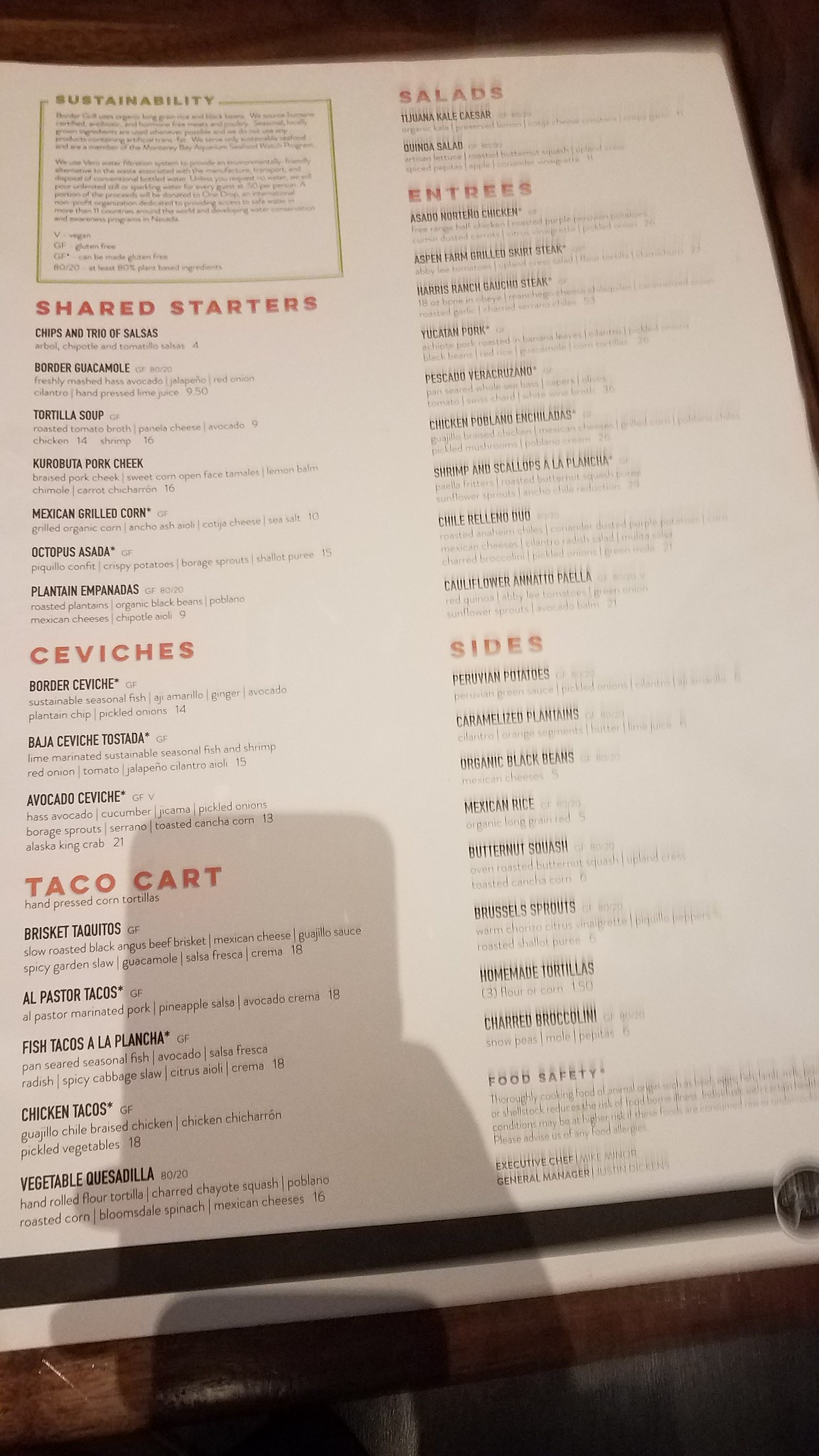The image features a long rectangular menu set against a solid black background, creating a striking contrast. The menu itself is white, adorned with a combination of red and black lettering, indicating various sections dedicated to shared starters, ceviche, taco cart, salads, entrées, and sides—suggesting it's from a dining establishment. In the lower region of the image, the shadow of the person holding and reading the menu is visible, adding a human element to the composition. There is also a black bar at the bottom of the menu, possibly as part of its design, though its specific purpose remains unclear. A partially obscured logo appears on the far right side of the image, though it is not legible. On the top left corner, a framed rectangular section contains a statement about sustainability, emphasizing the restaurant's commitment to eco-friendly practices.